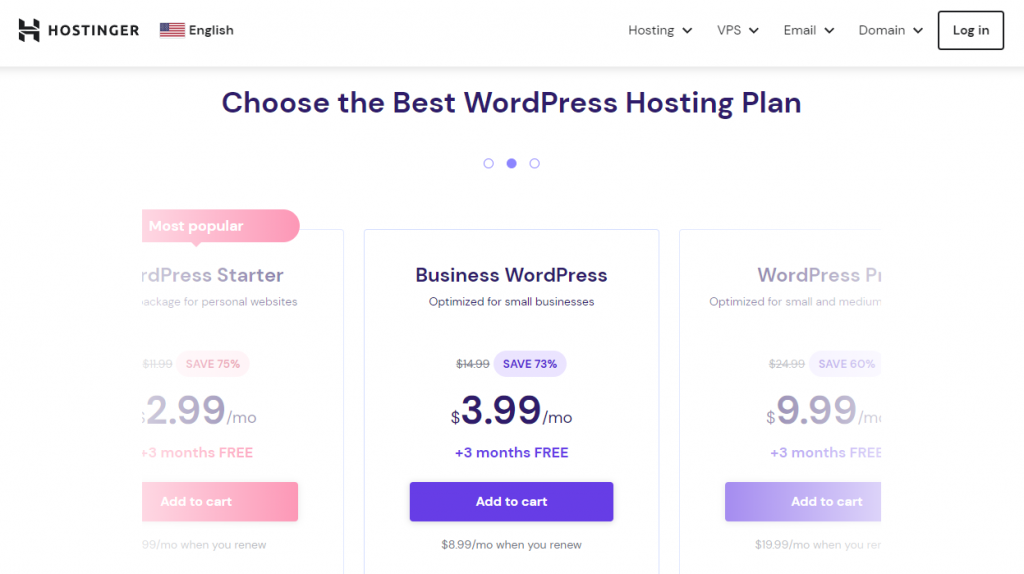The image is a webpage displaying WordPress hosting plans from Hostinger. The background of the page is white, and in the upper left corner, there is a bold black "H" emblem, followed by the bold black text "Hostinger." Adjacent to it is an American flag emblem in red, white, and blue, accompanied by smaller black text that reads "English."

To the right of this branding strip, there is a navigation menu with the following options: "Hosting" with a drop-down menu, "VPS" with a drop-down menu, "Email" with a drop-down menu, and "Domain" with a drop-down menu. In the far right corner of the header, there is a white rectangle with a black border containing the text "Log In."

Below the header, the main content begins with a prominent heading that says, "Choose the best WordPress hosting plan." Directly beneath this heading are three circles used for navigation. The center circle is blue, while the two on either side are white on the inside with blue borders.

To the left, within the body of the page, there are three distinct hosting plan options, each displayed within a square. The leftmost square has a red bubble at the top labeled "Most Popular." Below this tag, the plan is titled "WordPress Starter," described as a package for personal websites. The plan advertises a 75% savings at a rate of $2.99 per month, with an additional offer of three months free. At the bottom of this square, there is a red rectangle with white text that says "Add to Cart."

In the middle square, the plan is named "Business WordPress," optimized for small businesses. It offers a 73% discount, resulting in a monthly cost of $3.99, plus three months free. This plan also has an "Add to Cart" button at the bottom.

The rightmost square presents the "WordPress Pro" plan, optimized for small and medium businesses. This plan provides a 60% discount, priced at $9.99 per month, with an additional three months free. A blue "Add to Cart" button is located at the bottom of this square.